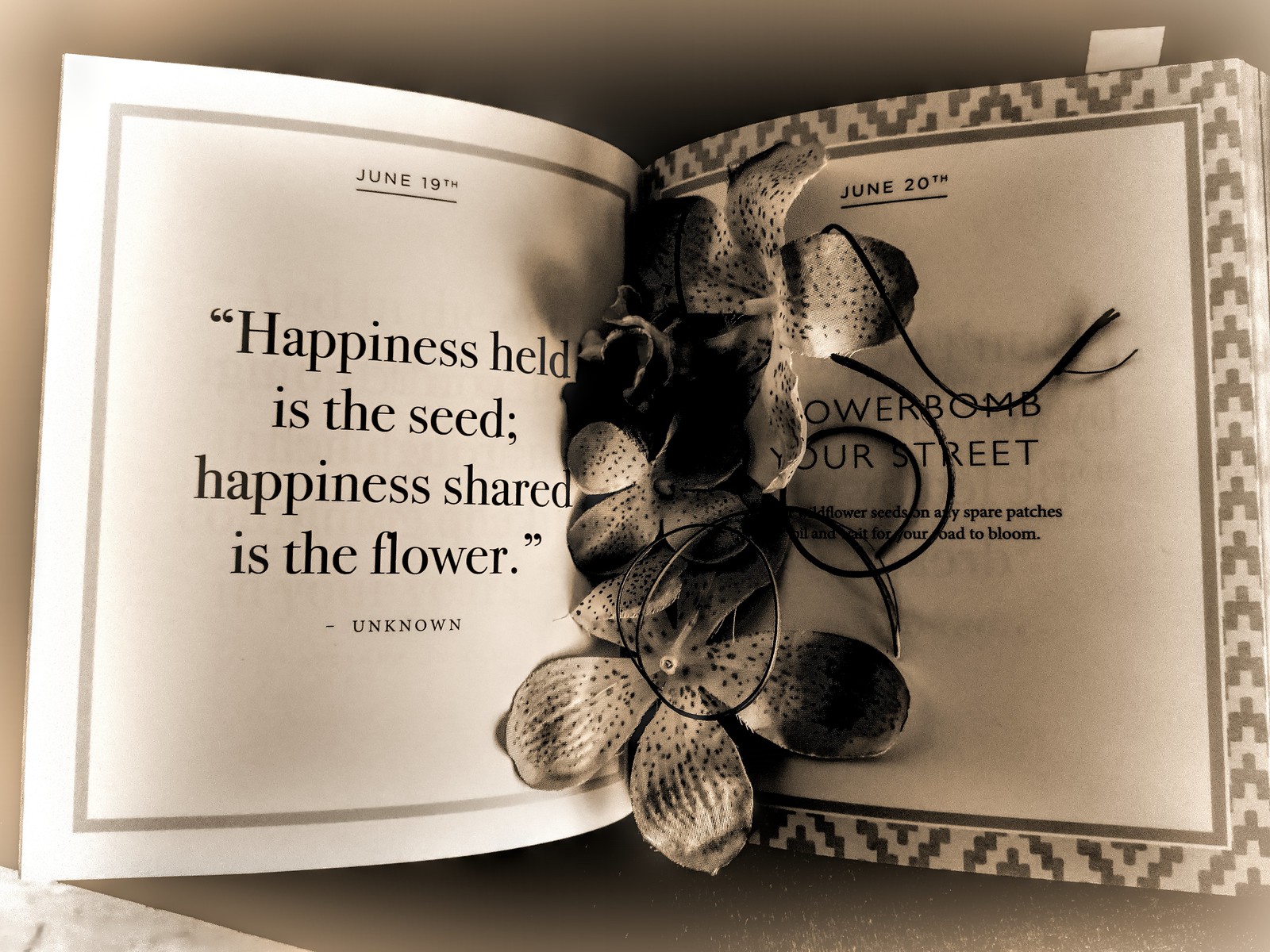The image features an open book lying on a grey surface. Down the center seam of the book, there are black and white floral illustrations, giving the impression that flowers are emerging from within the book. The left page is bordered with a decorative grey design and contains the black text: "Happiness held is the seed; happiness shared is the flower." The quote, attributed to "unknown," is positioned below an underlined date, June 19th. On the right page, there is also a patterned border, and it bears an underlined date, June 20th, followed by the phrase "Flower bomb your street" in black text. The bold floral motifs are prominent in the center, extending onto the right page, and while they appear large and five-petaled, they are illustrations rather than real or plastic flowers.